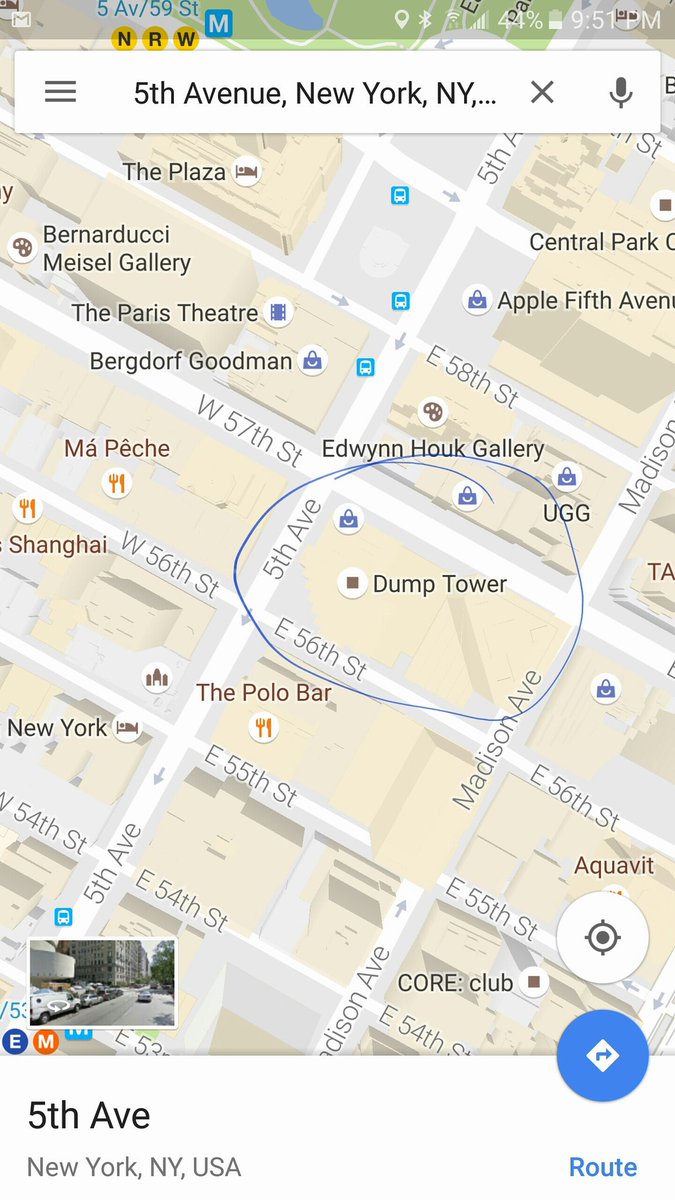Screenshot of a mobile map application displaying a detailed street grid at an angle. Dominating the display is Fifth Avenue, a straight road stretching from the bottom left to the top right, clearly labeled in black text. Crossing it at a 90-degree angle is West 57th Avenue, also prominently marked.

The map is dotted with various circular icons, each containing colorful emblems and labeled with black text outlined in white. At the top of the screen, there is a translucent black header featuring a white Gmail logo on the left. To the right of the logo are multiple white icons, further to the right, the time "9:51 p.m." is displayed.

Beneath this header sits a white search bar. On its left side are three horizontal gray lines stacked vertically, and typed into the bar is "Fifth Avenue, New York, New York,..." in black text. To the right within the search bar are a dark gray X and a dark gray microphone icon.

At the bottom right corner of the map are two prominent circular icons: a white circle with a dark gray reticle in the center, and a blue circle featuring a white diamond with a blue right-pointing arrow inside it. Below these, on a white background, the word "Route" appears in blue text. On the top left of the same white backdrop, "Fifth Avenue" is written in black text, with "New York, New York, USA" in light gray text beneath it.

Centrally located on the map, there is a white circular icon with a brown square inside. To its right, "Dump Tower" is labeled in black text, encircled by a blue-drawn pen-like line.